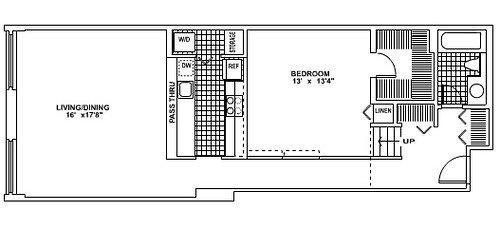The floor plan depicts a spacious layout with a variety of features and rooms. On the left side, there's a large rectangular border with ridged, stick-like shapes drawn into it. To the right of this border, a space is labeled "Living/Dining" and measures 16 feet by 17 feet, 8 inches. Adjacent to this area is a labeled pass-through, leading into a kitchen on the far right side.

In the upper left corner of the kitchen area, the letters "W something" denote an unspecified feature, with a storage room to its right, which contains a grid of squares in the center, possibly representing shelving or units. The left side of the kitchen is labeled "DW" (possibly a dishwasher), while the right side is designated for a refrigerator, with a sink and a stove situated between these appliances; the stove is illustrated with circled burners.

To the right of the kitchen is a bedroom, sized at 13 feet by 13 feet, 4 inches. This bedroom includes a closet with a swinging door, detailed with multiple lines indicating shelves.

Adjacent to the bedroom, a bathroom features a uniquely shaped bathtub, likened to a pinky pointing to the left. The bathroom also includes a grid of tiles and a sink. Below this area, there is another closet, indicated by lines and a swinging door at the bottom.

A staircase with small rectangular steps, labeled with an upward-pointing arrow, is noted next to the closet. There is also a large hallway running from the left side (starting from the living/dining area) to the right side where the staircase is located. A dotted line connects the staircase to the lower level of the floor plan, guiding the way to the down stairs.